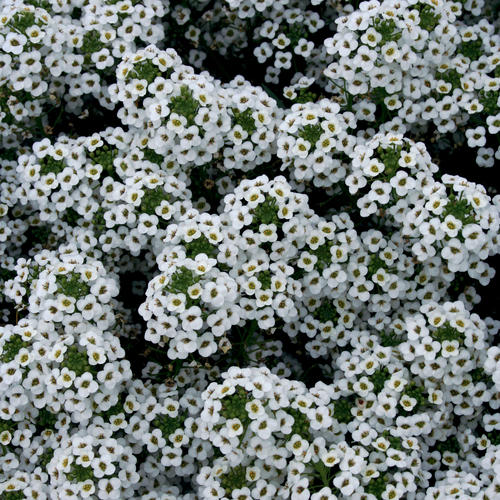The color photograph showcases a close-up view of numerous small white flowers, each featuring four rounded petals with a yellow center, forming distinct yet densely packed spherical clusters. The clusters dominate the image, covering much of the visible space, and are so densely packed that the green stems and leaves are only faintly discernible in some areas. Below and behind the clusters, the background is uniformly black, contributing to an isolated, almost spotlight effect on the flowers. There are no animals, people, buildings, or any man-made structures in the image, making the pristine clusters the sole focus of the scene.